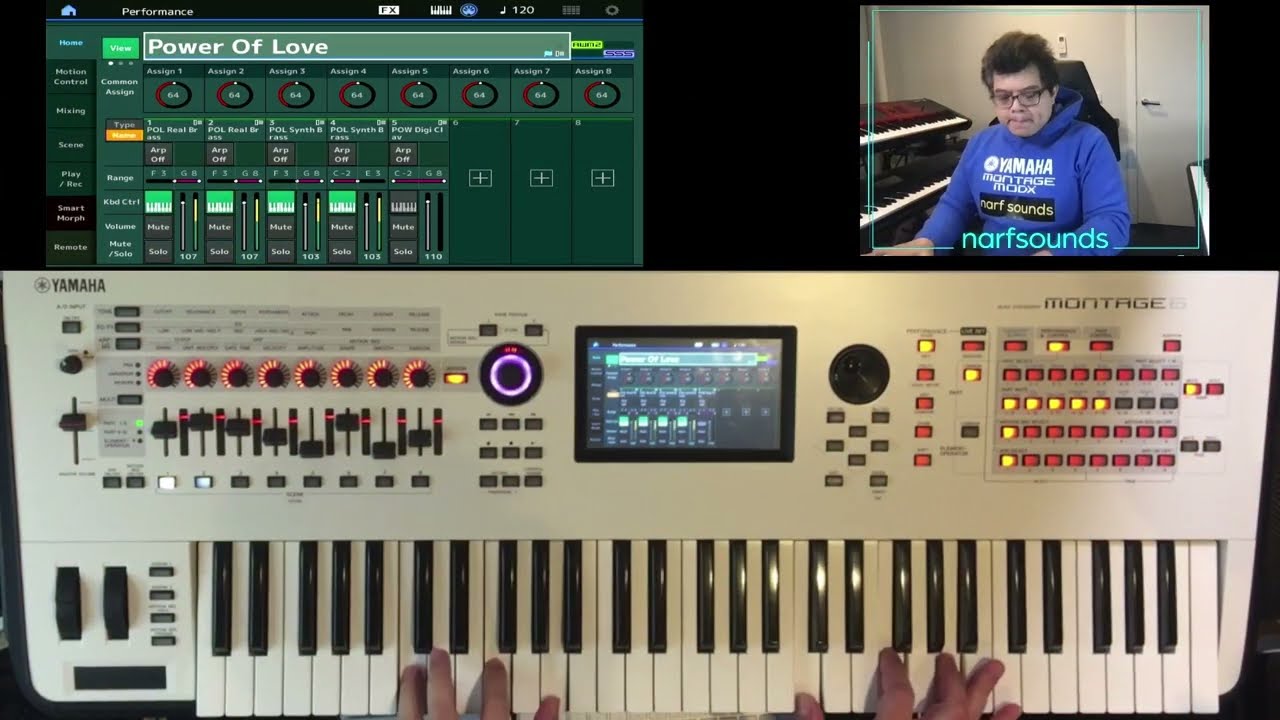The image showcases a composite arrangement featuring elements of a music production setting. In the lower half, a detailed view of a Yamaha Montage electronic keyboard is displayed, with human fingers actively playing on its ivory-colored keys. This keyboard is equipped with various controls, including numerous knobs and a small digital screen displaying adjustments, accented with red and yellow buttons.

In the upper left quadrant, an enlarged computer screen shows a digital sound mixing interface with the song title "Power of Love" prominently displayed. Adjacent to it, in the upper right quadrant, is a photograph of a middle-aged man with short, dark curly hair and black-rimmed glasses. He is wearing a blue hoodie branded with Yamaha and labeled "Narf Sounds," which also appears in green lettering below the image. The background reveals a white wall with a door and additional keyboards, suggesting a professional recording studio environment.